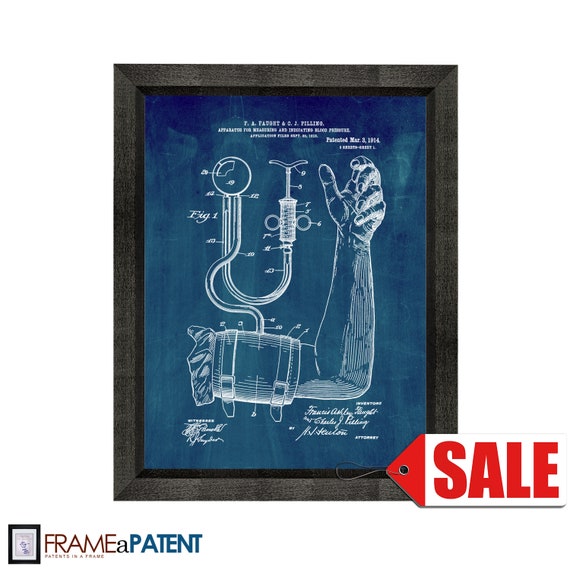The image appears to be a digital advertisement for the company "Frame a Patent," showcasing a framed blueprint of an old patent. The frame is dark grey or black and encloses a detailed, chalkboard-like drawing of a person's arm in a right-angle position. Wrapped around the upper arm is a vintage blood pressure cuff, connected by tubes to a measuring gauge and a syringe-like plunger. The diagram includes labeled components, though the text is too small to be legible. A date in the top right corner of the drawing indicates the patent was issued on March 3rd, 1914, and the title suggests it is an apparatus for measuring blood pressure. Additionally, a red and white sale tag lies near the bottom right of the image, while the company logo, "Frame a Patent," is placed in the bottom left, emphasizing the service of framing patent designs.